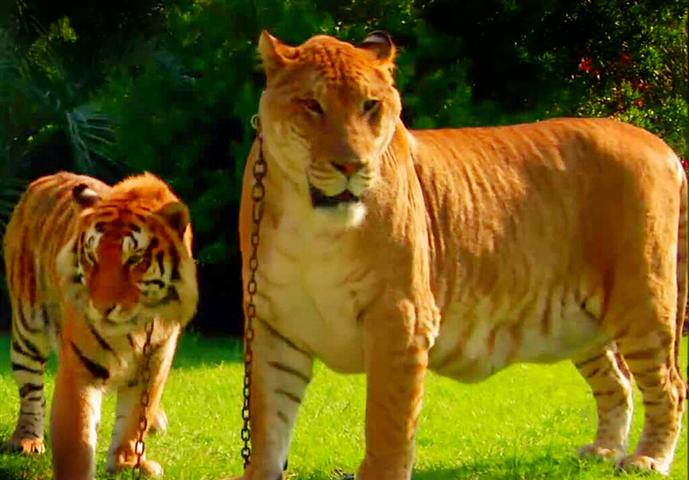In this outdoor scene, two felines are standing on well-manicured, vibrant green grass, surrounded by lush, deep green trees and some red flowers to the right. It's a sunny day. On the right stands a very large tiger with a striking golden-red body, adorned with subtle stripes along its legs and a white underbelly. This big male, with short, pointy ears and a wide facial structure, looks off to the side, his neck encumbered by a black chain that cascades down, evoking a sense of sadness. On the left, a much smaller tiger, possibly a cub, shares a similar chain around its neck. This smaller tiger has a more prominently striped body and face, with a solid red face featuring short, pointed ears, and it gazes in the opposite direction. Both animals are showcased in this natural yet somber setting, their majestic presence contrasted by the restricting chains they wear.